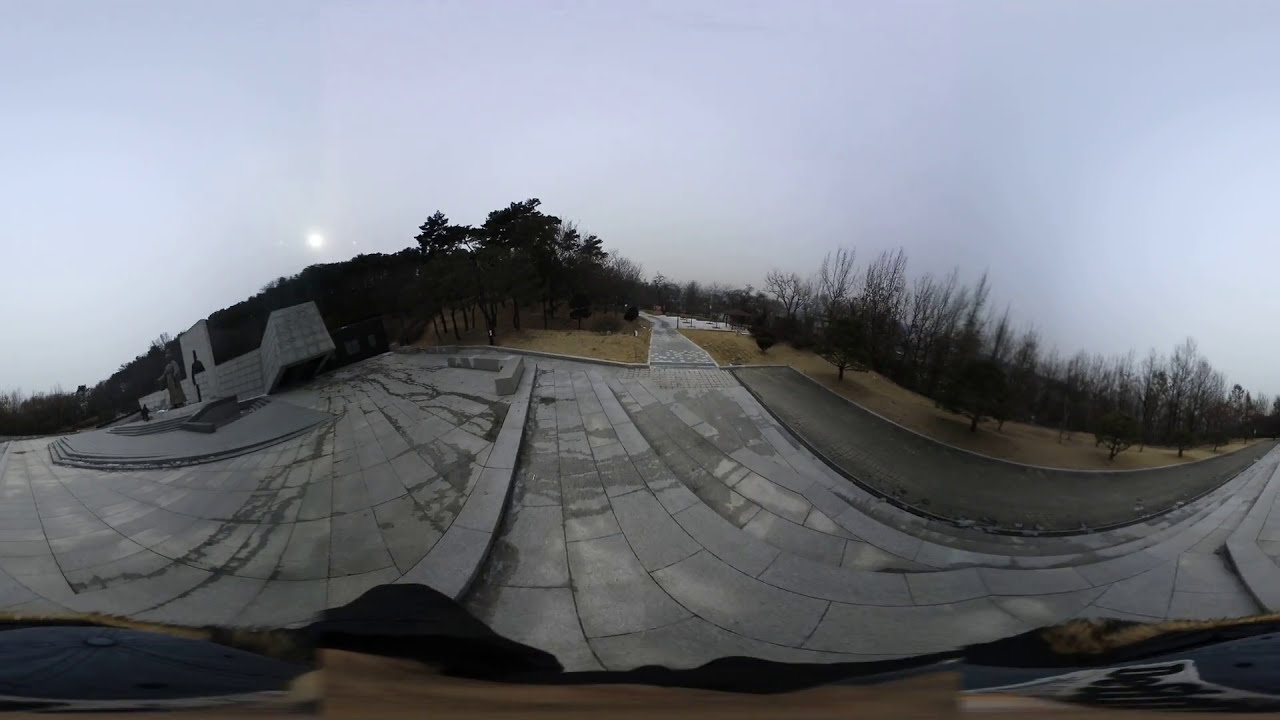This photograph captures a gray, overcast day at an outdoor park dominated by a significant monument. The scene is dimly lit, indicating it might be during the fall or winter, as the trees in the distance are barren and the grass is brown and dead. The focal point is a large granite-paved walkway, composed of sizeable gray stone blocks, that leads directly towards the monument positioned on the left side of the photo. This monument features multiple steps ascending to it and is flanked by stone structures. Beyond the monument, a wooded area with leafless trees is visible. The setting is enhanced by the absence of color vibrancy, contributing to the overall gloomy atmosphere.